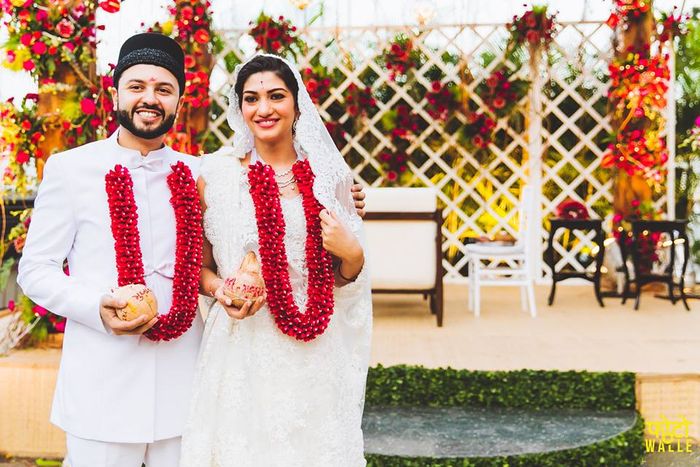This photograph depicts an Indian couple, perhaps during a wedding ceremony, positioned on the left side of the frame. Both are adorned in traditional attire; the man wears a white suit complemented by a black cylindrical hat and sports a neatly trimmed black beard. The woman is dressed in an off-white wedding dress complete with a flowing veil. They each have a distinct mark on their foreheads: the man has a red thumbprint-like mark, while the woman features a forehead gem. Both are adorned with thick, dark red flower leis that drape from their chest level down to their waists. In their right hands, they are holding uniquely shaped vegetables—he has a round one, and she holds an elongated pear-shaped one. The background showcases a beautifully decorated patio with white latticework interwoven with vibrant red flowers and surrounded by a variety of white and black patio furniture, including chairs, benches, and stools. Directly behind them lies a serene water pond encircled by lush green vegetation.